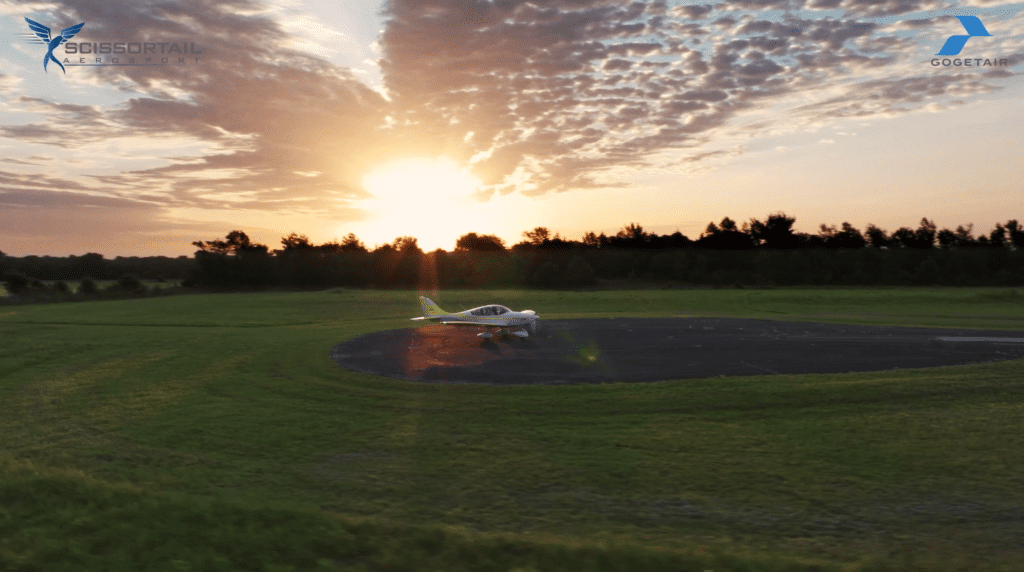The photograph captures a landscape at sunset featuring a small silver and gray airplane that has landed in the middle of a grassy field, designated as a landing area. The vibrant sky is a blend of blue, peach, and light shades of orange and yellow, with the Sun casting its rays amidst gray cloud formations. The background is adorned with the black and brown silhouettes of trees. Positioned horizontally, the center of the image is dominated by the airplane, albeit somewhat obscured by the bright sunset that overpowers the photo. In the upper right-hand corner, two blue logos are visible: one reads "Scissortail Airport" and the other "Gogetair." The photograph is well-lit with natural lighting and, despite its clarity, lacks a professional touch. Overall, the image vividly captures the serene yet dynamic essence of an outdoor sunset setting.